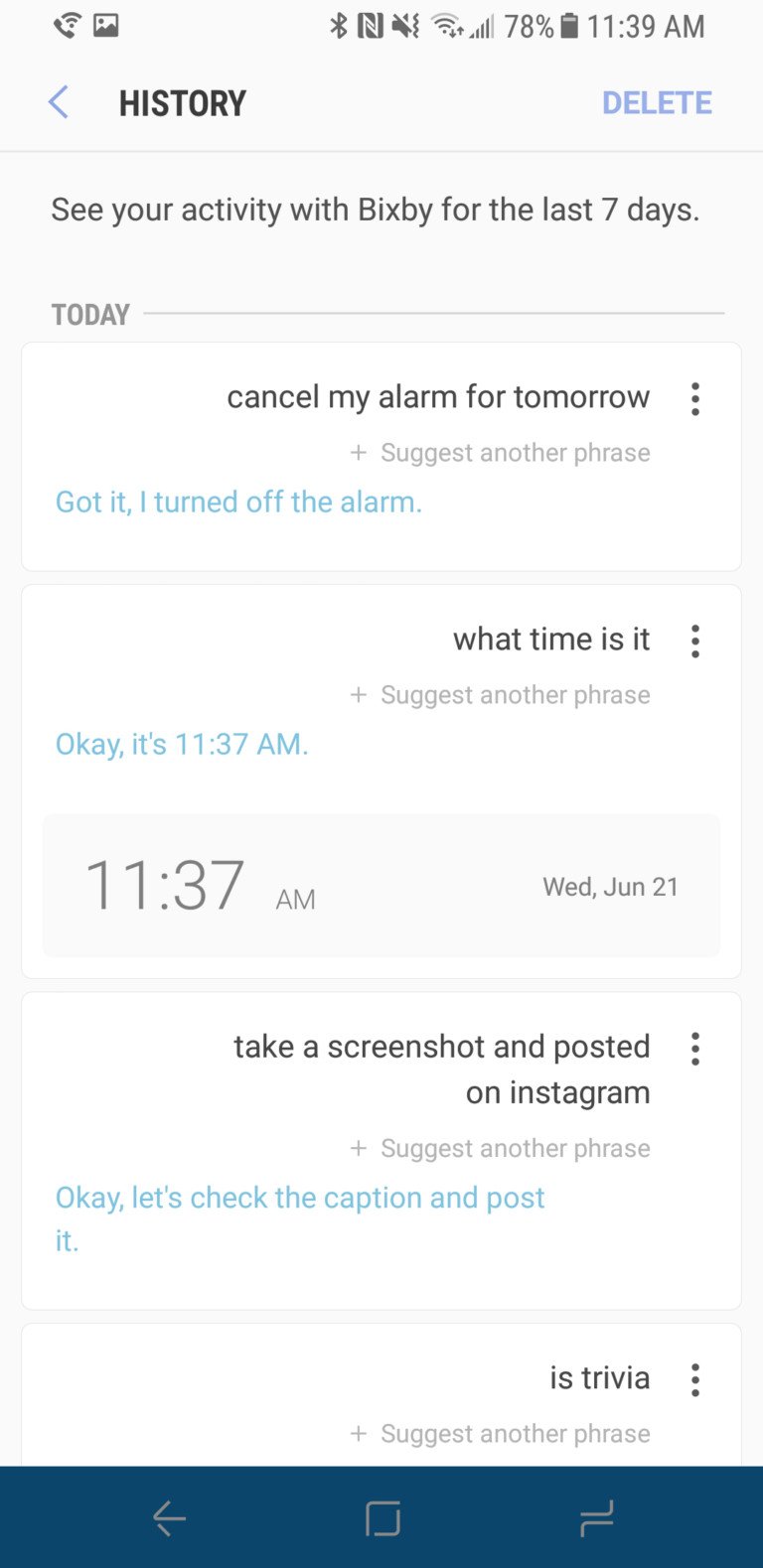The image, captured on a cell phone screen with a battery life of 78% at 11:39 AM, displays a user interaction with Bixby. At the top left corner, a small blue arrow points to the left beside the bold black text "History." To the right, there's the blue option labeled "Delete." The screen shows Bixby's activity over the last seven days. Today, indicated by a long light gray line, features commands like "Cancel my alarm for tomorrow," followed by an icon with vertical circles labeled "Suggest another phrase."

Bixby's response is highlighted in blue reading, "Got it. I turned off the alarm." Below, the user asks, "What time is it?" and Bixby responds again in blue text, "OK, it's 11:37 AM." The timestamp, 11:37 AM, appears in gray with the date "WED, June 21" to the right.

Further down, another command reads, "Take a screenshot and post it on Instagram," to which Bixby replies in blue, "OK, let's check the caption and post." At the bottom of the screen, there is a long blue rectangle with an embedded arrow pointing left and a square inside, representing another interactive element of the interface.